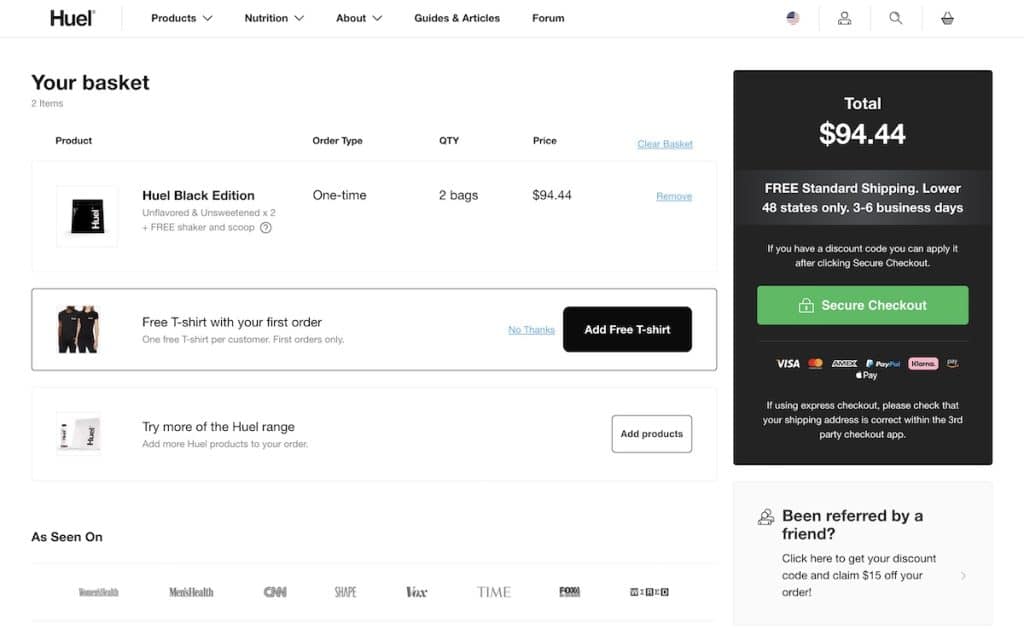Here is a cleaned-up and detailed caption for the image described:

---

The image depicts an order screen on the Huel website, characterized by a clean white background. In the upper left corner, "Huel" is prominently displayed in bold black letters. Adjacent to it, in a slightly less bold font, are navigational tabs including Products, Nutrition, About, Guides & Articles, and Forums. Moving to the right, there are icons for an American flag, a user profile, a search function, and a shopping basket.

Below this header, the main section reads "Your Basket: 2 items." The basket's details are organized into categories: Product, Order Type, Quantity, Price, along with a Clear Basket button. Listed in the basket are: "Huel Black Edition, Unflavored and Unsweetened" (2 bags), with a promotional offer of a free shaker and scoop. The price for these items is $94.44. An additional offer for a free T-shirt is available, but only for first-time customers, with options to decline or add the T-shirt.

Further down, promotional encouragement suggests adding more Huel products, endorsed by publications such as Men's Health, CNN, Shape, Vox, Time, Fox Business, and Wired. 

On the right side, in a prominent black box, the total price of $94.44 is displayed, accompanied by details about free standard shipping to the lower 48 states (estimated delivery within 3-6 business days). It also mentions the option to apply a discount code after proceeding to checkout. The checkout process can be initiated by clicking the green "Secure Checkout" button featuring white text.